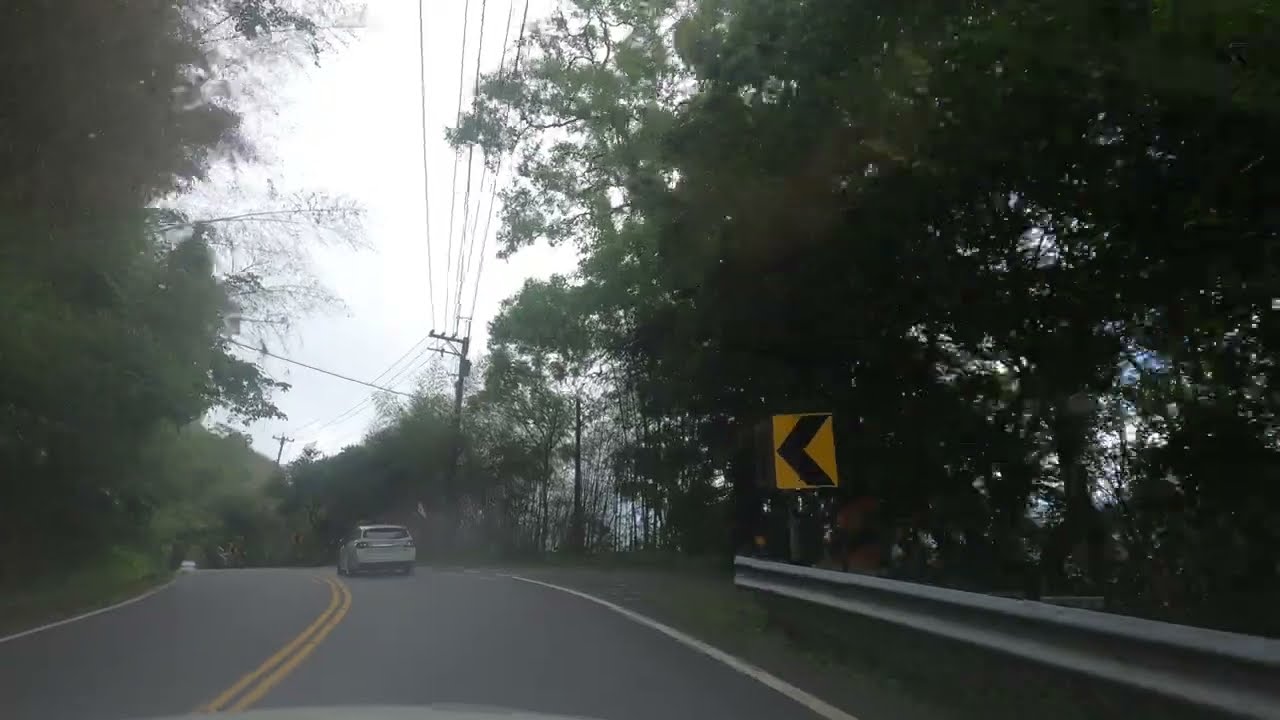This horizontally aligned, rectangular photograph, likely taken from inside a vehicle through a windshield, presents a slightly blurred view of a rural two-lane road. The road is defined by double solid yellow lines in the center and white lines segregating the shoulder. A gray or white sedan can be seen driving away from the observer. In the lower right corner, a metal guardrail and a rectangular yellow traffic sign with a black arrow indicating a leftward curve highlight the foreground. The image captures numerous utility poles with power lines lining the right side of the road, set against a backdrop of abundant green foliage on both sides. The road itself appears to curve to the left in the middle distance, with trees densely populating both sides, and a small hill is visible further ahead. The sky above is overcast with a mix of bright white, gray clouds, and occasional patches of blue peeking through the branches. The scene conveys the feeling of an open, country roadway on a cloudy day.